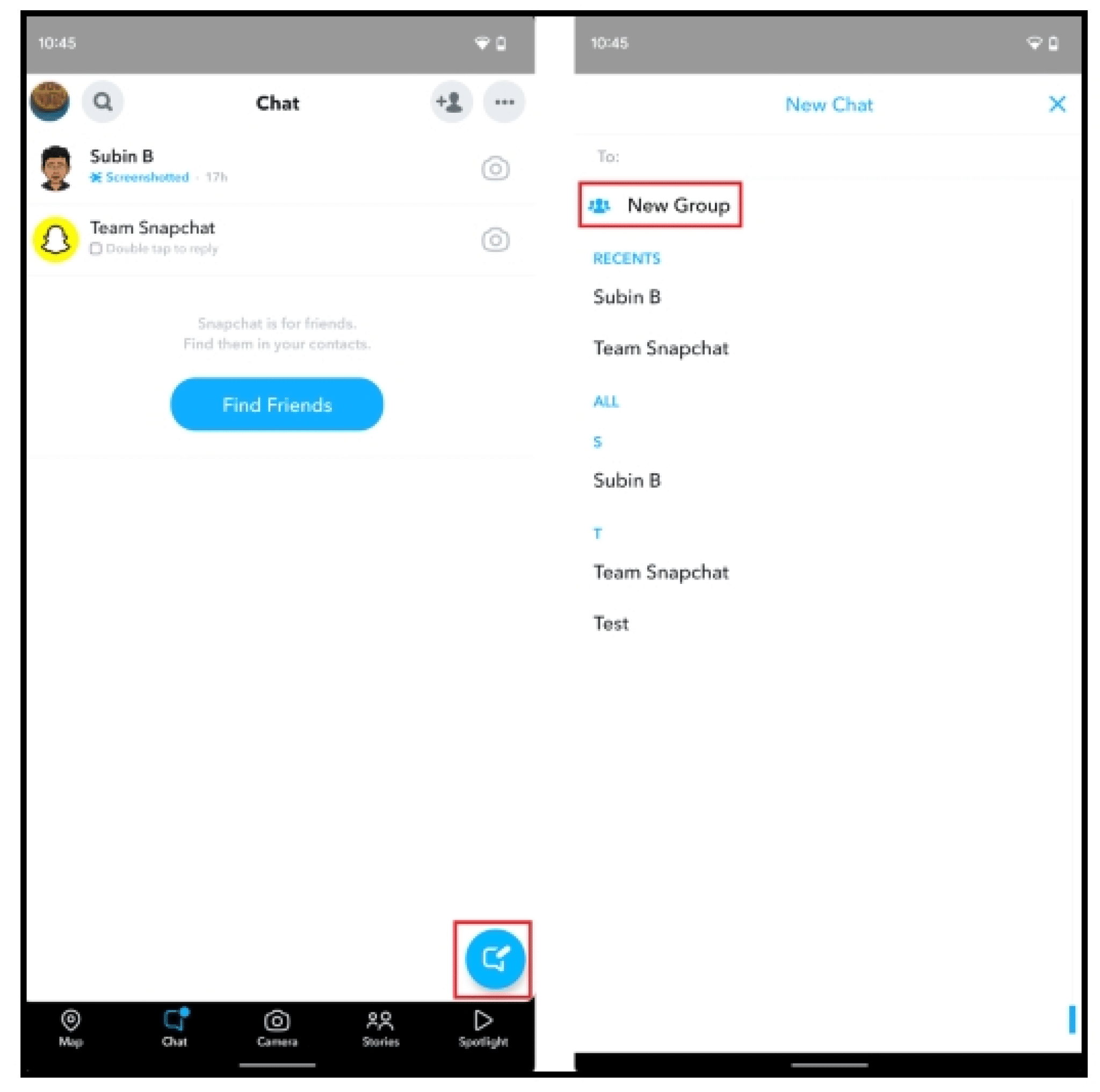The image is a side-by-side view of two smartphone screenshots, each framed within a square shape with a black border and separated by a white bar in the middle. Both screenshots display the current time as 10:45 at the top left corner, alongside Wi-Fi and battery indicators at the top right.

On the left screenshot, the interface appears to be a messaging or social media app. At the top left is a circular profile icon, next to a circular search bar. Centrally, the word "Chat" is displayed. To its right, there is an icon of a person with a plus sign and a three-dot menu icon for additional options. Below, a circular picture icon is followed by a name and some blue text, likely a username or status, with a camera icon on the far right. Further down, there is a notification symbol with a yellow circle indicating "Team Snapchat" and another camera icon to its right. The most prominent feature on this side is a large blue button labeled "Find Friends," and beneath that, at the bottom right, a circular icon enclosed in a red square is visible, all resting above the standard phone navigation bar.

The right screenshot predominantly features a white background with blue and black text, though specific content details are not clear. The overall composition suggests it might be part of a conversation or a different segment of the app shown in the left screenshot.